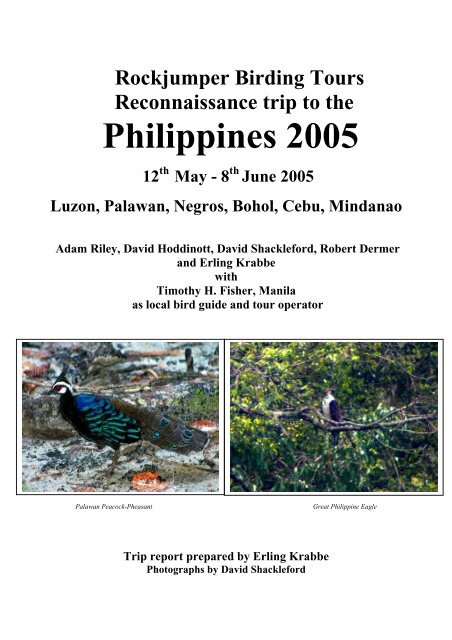This poster advertises Rockjumper Birding Tours' Reconnaissance Trip to the Philippines, held from May 12th to June 8th, 2005. The tour covers various locations, including Luzon, Palawan, Negros, Bohol, Cebu, and Mindanao. The design features two bird photographs captured by David Shackelford. On the left, a close-up of a Palawan peacock-pheasant showcases its intricate blue neck feathers, green wing feathers, black chest, and long light brown tail, with distinctive white facial markings and a red eye. On the right, a great Philippine eagle perches on a tree branch against a backdrop of lush green leaves, displaying a white chest and black feathers on its head. Below the images, the text credits Erling Krabbe for preparing the trip report, with local guide and tour operator Timothy H. Fisher based in Manila. The poster is detailed with names of key individuals involved, including Adam Riley, David Hoddinott, Robert Dermer, and Erling Krabbe. The professional and concise black text is set against a clean white background.